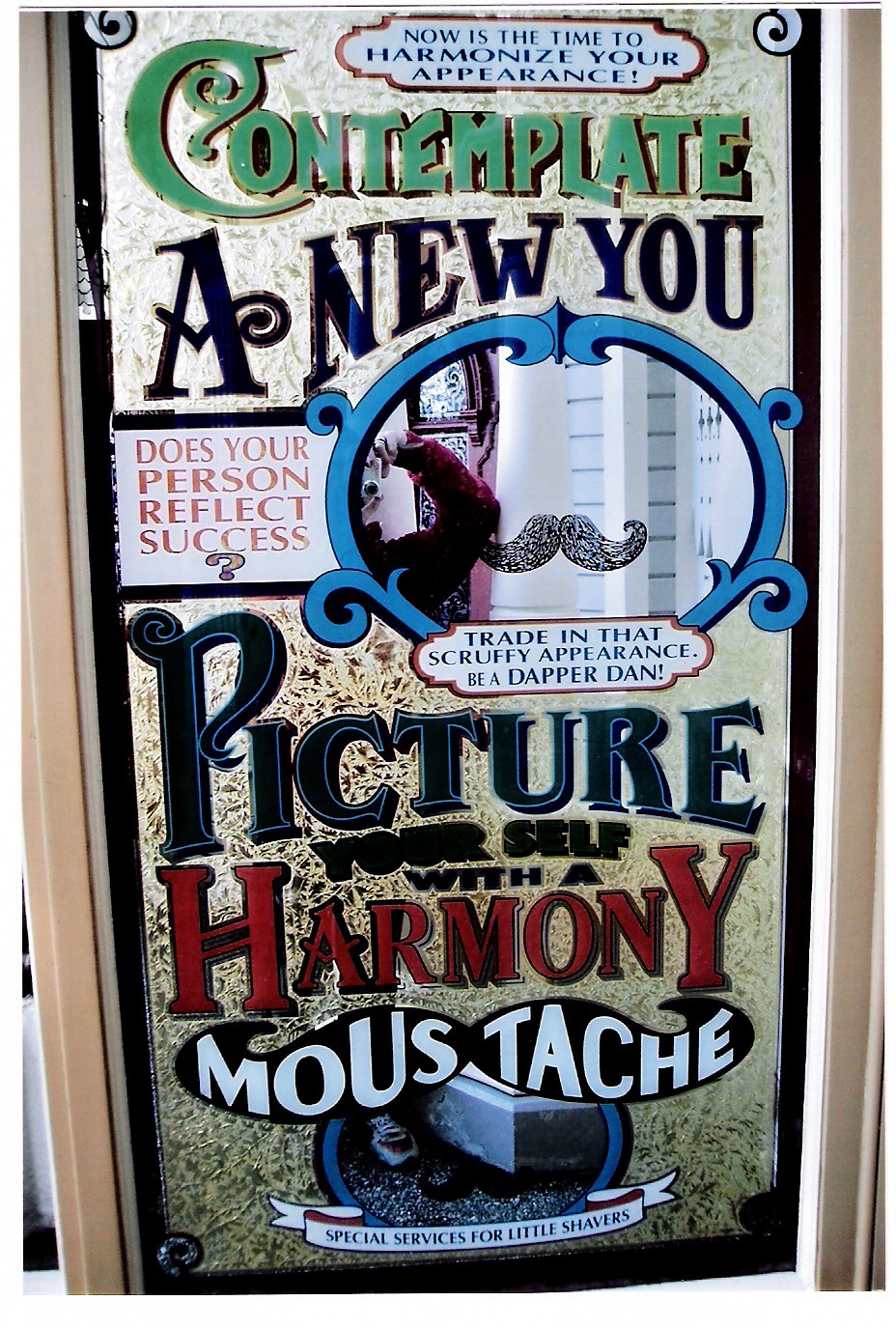This vibrant and whimsical photograph captures a creatively designed vintage-style banner, displayed in a shop window. The close-up image reveals the elaborate details of the colorful advertisement for a 'harmony mustache.' Set against a white background, the nostalgic font headlines with, "Now is the time to harmonize your appearance." Below, green and black text reads, "Contemplate a new you," followed by, "Does your person reflect success?" Centered in the banner is a striking blue circle featuring a handlebar mustache illustration. Further messaging urges viewers to "Trade in that scruffy appearance. Be a dapper Dan." In dark blue letters, "Picture yourself with a" is printed above the word "harmony" in vivid red, and "mustache" in bold white letters superimposed on a black mustache outline. At the bottom, within a white-bordered ribbon, the sign offers "Special services for little shavers." The design cleverly allows tourists to pose behind a transparent glass plate adorned with the mustache, creating an amusing photo opportunity where they appear mustachioed. The playful installation serves as both an advertisement and an engaging attraction for all ages.